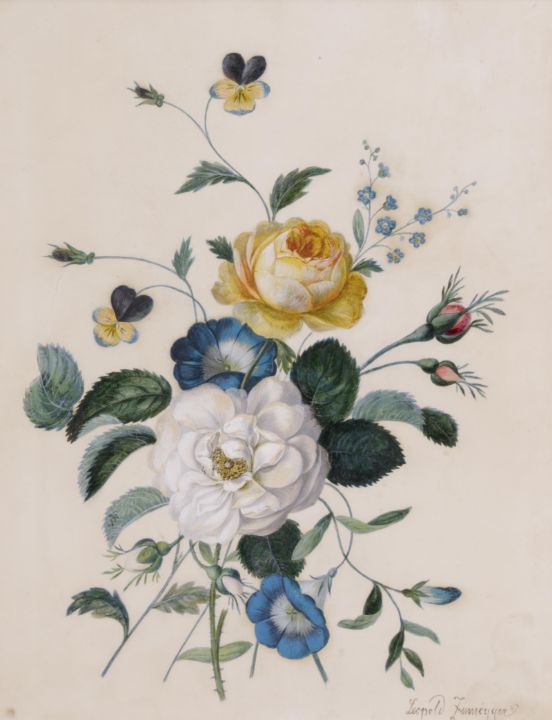This is an illustration, likely created with paint or watercolor, depicting a loose bouquet of vibrant flowers set against a cream-colored background. Dominating the center is a large white flower with pristine petals, surrounded by spiky green leaves. Immediately above and slightly below this focal point are striking flowers with white centers and blue outer petals. Above these blooms is a partially opened yellow flower, adding to the dynamic composition. To the right, there are what appear to be budding roses, while smaller flowers and additional foliage extend to the left and top of the image. Various green stems and slender leaves add depth and complexity to the arrangement. The entire piece has a slightly aged, stained appearance, suggesting it may have been created some time ago. At the bottom right of the canvas, there is a barely legible cursive signature, presumably that of the artist.